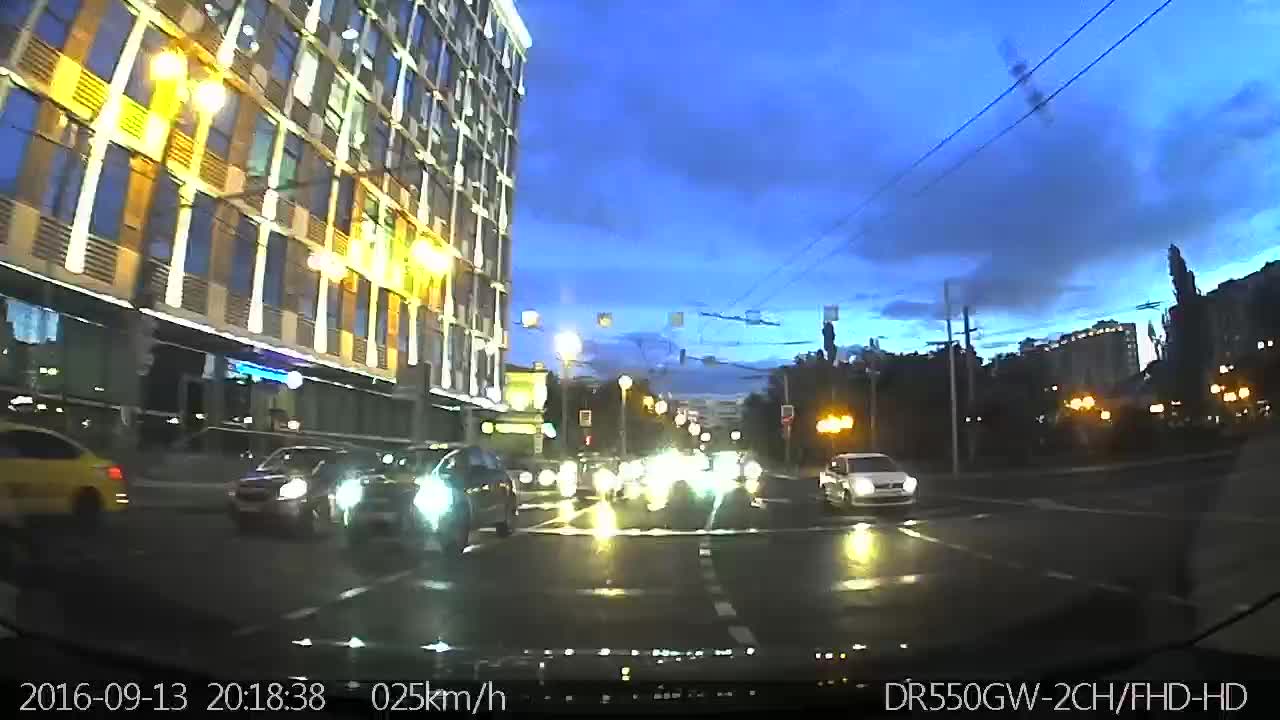In this outdoor color photograph taken at either dusk or dawn, the rear window of a car provides a wide-angle perspective, capturing a city street scene with a horizon approximately halfway up the image. The sky is a deep blue, transitioning to an aquamarine hue with light clouds scattered across. The street, which appears to be four to five lanes wide, is filled with oncoming traffic. Headlights from the numerous vehicles create a blur of white spots, though three four-door sedans on the left and one on the right are distinctly visible. Notably, a silver SUV and a yellow taxi with black writing can be identified among the cars. A prominent six to seven-story building with rectangular windows and silver columns occupies the left of the center, extending towards the upper right corner. Glowing yellow street lamps stand in front of this building, enhancing the scene. Street markings in the foreground show white dashed lines. In the lower left corner, a timestamp reads "2016-09-13 20:18:38" followed by "025 KM/H" and the camera model "DR550GW-2CH-FD-HD" indicating this may be a dashcam image.